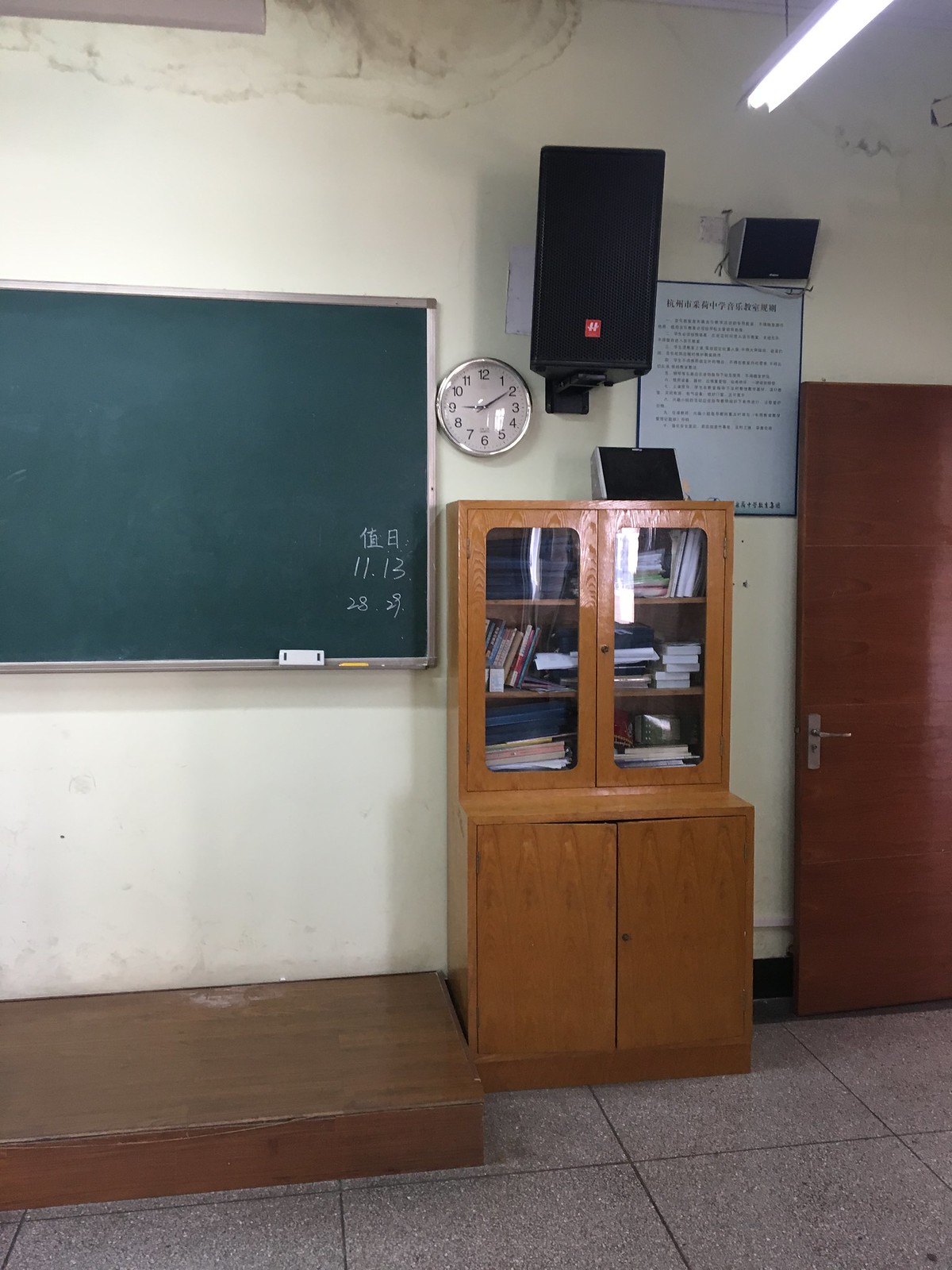A detailed photograph of a classroom presents a rectangular frame where the left and right sides are longer than the top and bottom edges. The photo prominently features large gray tiles with black grouting, adorned with various white and black specks, covering the floor in the bottom section of the image. In the bottom left corner, a raised wooden platform partially appears, crafted from brown-stained wood, and positioned against a white wall with a black baseboard. Above the platform, a green chalkboard with a silver metal frame occupies a section of the wall. The chalkboard includes a small lip or shelf at the bottom edge, upon which rests a small rectangular white eraser and a white stick of chalk on the right side. The chalkboard also features some writing, though the specifics are not detailed in the description.